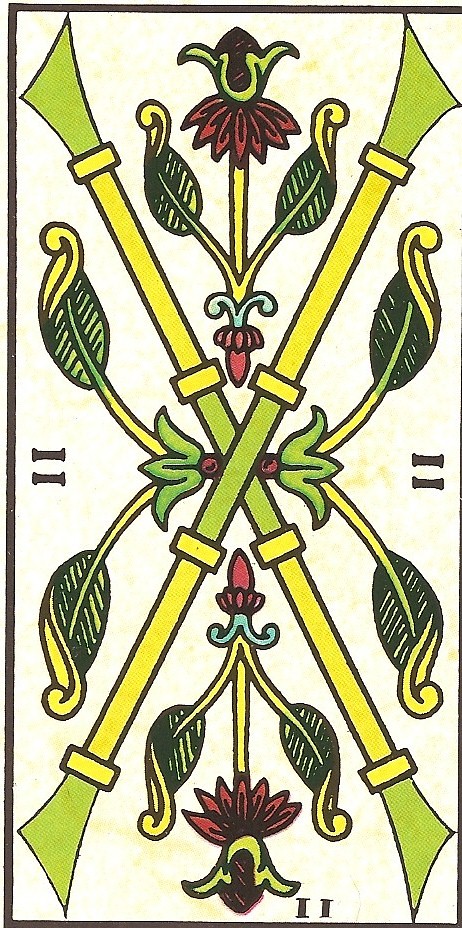The image appears to be a high-resolution scan or a computer-generated depiction of an intricate artwork. The centerpiece is a large, prominent "X" shape formed by two intersecting bars: one extending from the top left to the bottom right, and the other from the bottom left to the top right. These bars comprise alternating sections of yellow and green cylinders, with yellow perpendicular crossbars dividing each section.

Nestled at the precise intersection of the "X" are two striking red circles outlined in black. Extending from the sides of the "X" is a green plant-like motif encased by yellow stalks. These stalks branch outwards with two extending upwards and two downwards. Each stalk culminates into leaf shapes adorned with horizontal black cross patterns and twist-like yellow infills.

Additionally, at both the top and bottom ends of the central design, similar leaf-stalk patterns emerge, enhancing the artwork's complex and symmetrical nature. The overall visual impression is one of dynamic movement and intricate structure, blending geometric precision with organic elements.